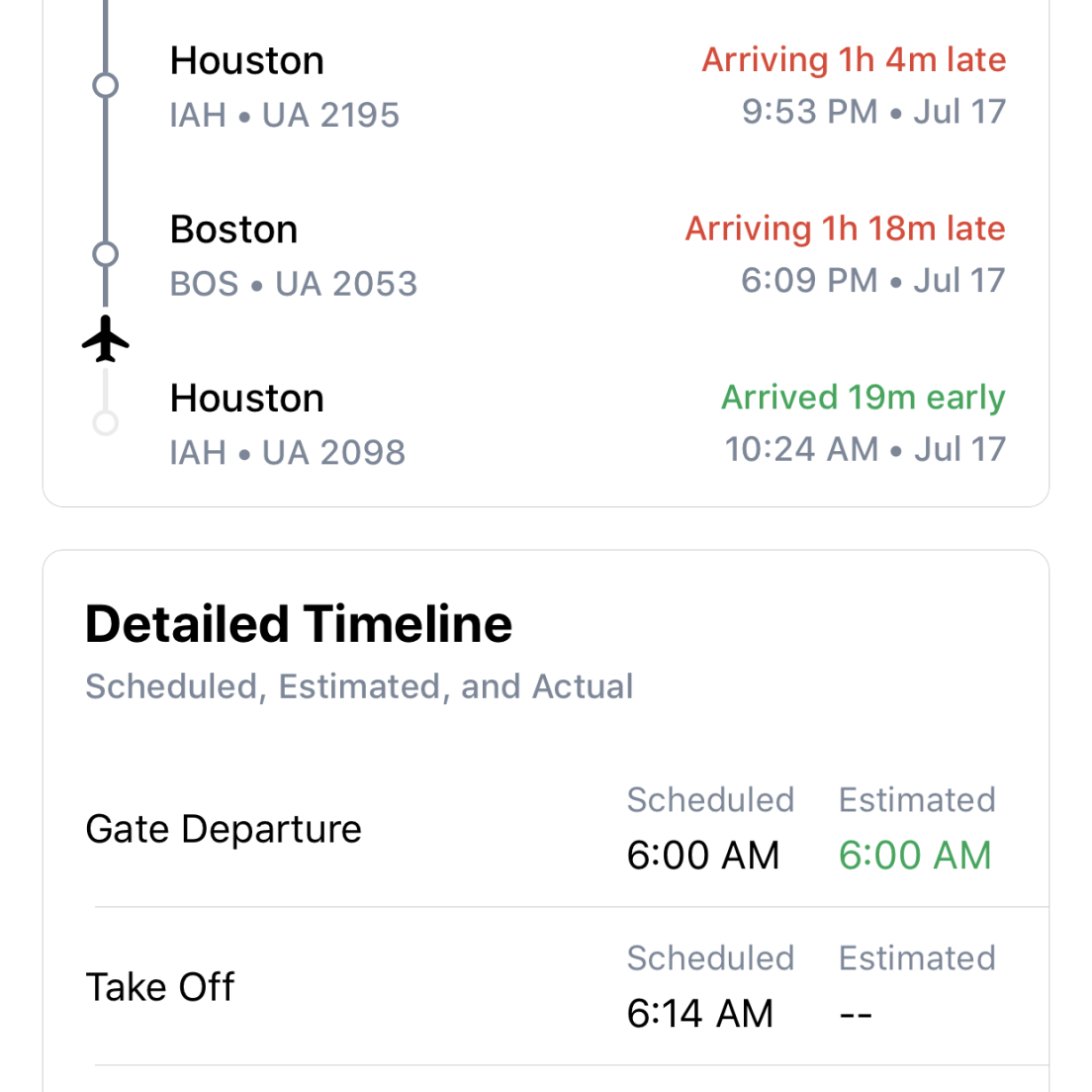A vertically-oriented computer or laptop screen displays detailed flight schedule information against a white background. The text, mostly in black, highlights the status and timings of a round trip that began in Houston, subsequently heads to Boston, and returns to Houston.

- **Houston Arrival:** The flight arrived 19 minutes early at 10:24 a.m. on July 17th.
- **Boston Arrival:** Scheduled to arrive at 4:51 p.m., this leg is delayed, now expected at 6:09 p.m., one hour and 18 minutes late.
- **Return to Houston:** Initially scheduled for a later time, it is now projected to arrive at 9:53 p.m., one hour and four minutes late on the same day.

Beneath this information, a separate section labeled "Detailed Timeline" in black letters contains subheadings in gray for "Scheduled," "Estimated," and "Actual" times:
- **Gate Departure:** Scheduled and estimated times both listed as 6:00 a.m.
- **Takeoff:** Scheduled for 6:14 a.m., but estimated time is not provided and is marked with two dashes.